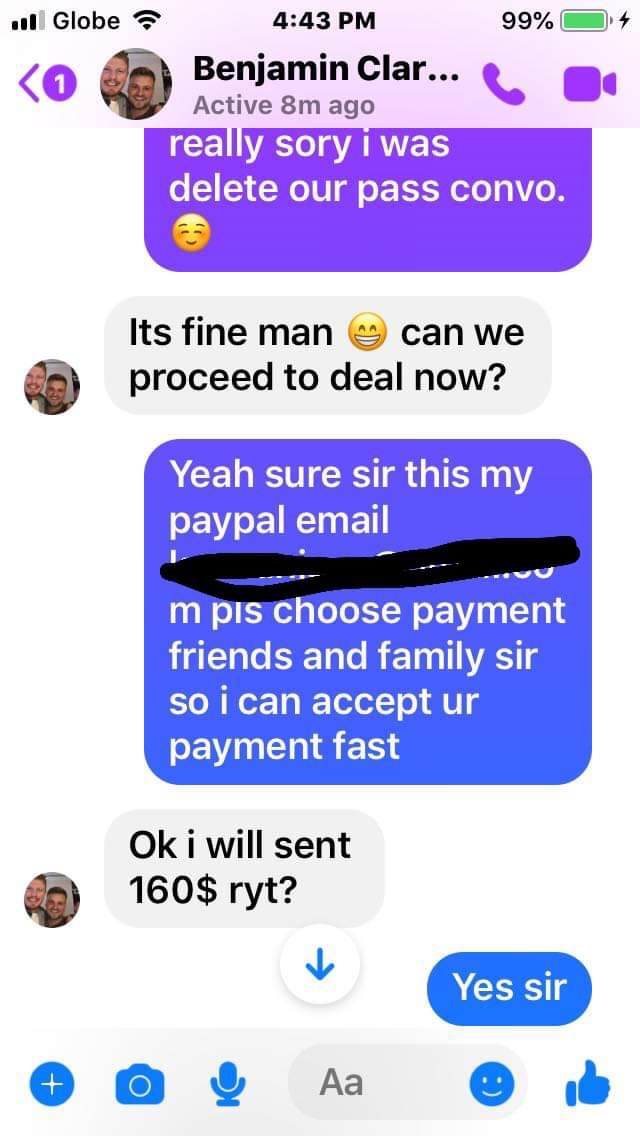This is a detailed description of a text message conversation, likely from a messaging app like Facebook Messenger, displayed on an iPhone screen with a white background. At the top of the screen, there's a status bar showing a signal strength of three out of four bars, the carrier name "GLOBE," a Wi-Fi icon, the time "4:43 PM," and a battery indicator showing 99% with a charging symbol. Below this, to the left, is a purple arrow indicator and a purple circle with the number one inside it. Adjacent to these is a circular profile picture of two men, associated with the name "BenjaminClark...," followed by purple icons for a phone and video call. In a purple speech bubble, Benjamin starts with, "Really sorry, I was delete our press convo," and includes a blushing smiling face emoji. The replying message in a gray bubble reads, "It's fine man 😊, we can proceed to deal now." Following this, in a dark blue rounded-edged bubble, the conversation continues with, "Yes, sure sir, this is my PayPal email," which is partially redacted, and "Please choose payment friends and family sir so I can accept your payment fast." Benjamin then replies in another gray bubble, "Okay, I will send $160, right?" with the final confirmation, "Yes, sir," in a blue bubble. At the bottom of the screen, the interface shows several blue icons for composing messages: a plus sign, a camera, a microphone, a text input area with "Aa," a smiley face, and a thumbs up.